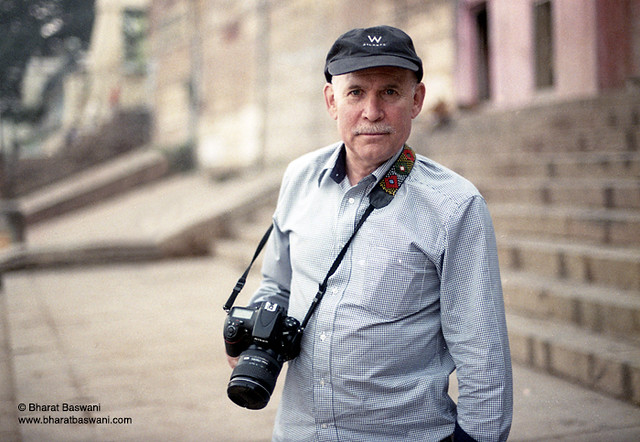The image features a close-up photograph of an elderly man, approximately 60 to 65 years old, standing outdoors next to an old, large brick building, likely bathed in daylight. The man has light blue eyes, a gray mustache, and very short, thin eyebrows. He sports a black baseball cap with a white 'W' emblazoned on the front and is dressed in a textured blue and white long-sleeved dress shirt with a front pocket. The shirt is buttoned down and not tucked in. Around his neck hangs a professional DSLR camera on a strap that is red, white, and black. He holds the camera in his right hand, while his left hand appears to be near or in his pocket. The background is slightly blurred but reveals cement blocks and sunlight. In the bottom left corner of the photograph, there is a watermark that reads "© Bharat Baswani" with the website "www.bharatbaswani.com."